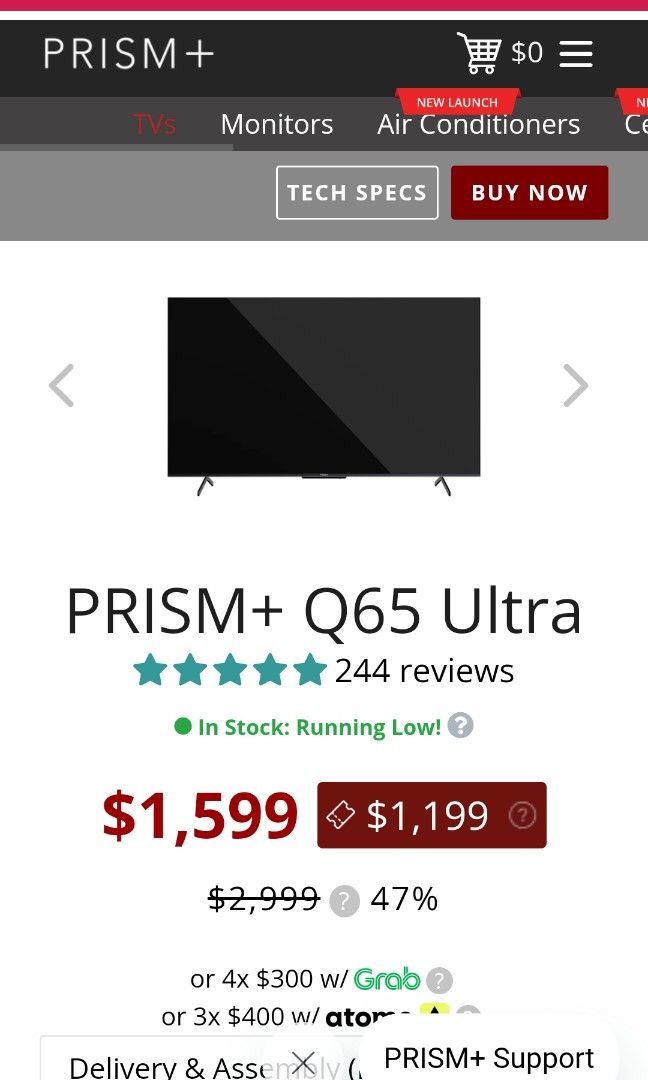At the top of the page, a thin red rectangle bar spans across the width. Directly beneath this, a black rectangle with bold white text prominently displays "PRISM PLUS". Adjacent to this, a white icon featuring a shopping cart with a dollar sign is accompanied by the number zero.

Below the black rectangle, a gray bar is situated, featuring the word "TVs" in red text and "Monitors" in white text. Encased in a white-outlined rectangle within this gray bar, the term "Tech Specs" is also written in white. Additionally, a red rectangle with the phrase "Buy Now" in white lettering is presented.

A central image showcases a TV, flanked by left and right arrows. Beneath this image, the product name "PRISM PLUS Q65 Ultra" is highlighted. Accompanying this, five blue stars and the text "244 reviews" signify customer feedback. A small green dot is paired with the gray text "In Stock, Running Low," indicating the product's availability. The price, highlighted in vivid red text, reads $1599. A small gray circle featuring a question mark appears for additional information.